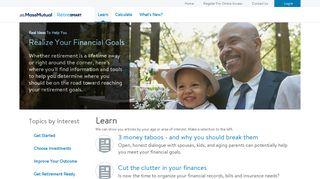A blurry, small image appears to depict a financial advice webpage. If viewed on a minimized laptop screen or a phone turned sideways, the text is difficult to decipher. The header reads "Realize your financial goals" in the top left corner, followed by a section titled "Topics by Interest." Despite the blurriness, some of the article titles in blue writing can be made out: "Learn three money taboos and why you should break them" and "Cut the clutter in your finances." There’s a black area on the right side of the screen with contrasting white text. Further to the right, a man wearing what seems to be a black jacket or vest over a white shirt and black tie is seated with a child in his lap; the child, donning a hat, is nestled comfortably. Nearby, part of another person’s shoulder is faintly visible. The background features trees and flowers, lending a natural setting to the otherwise informational scene.